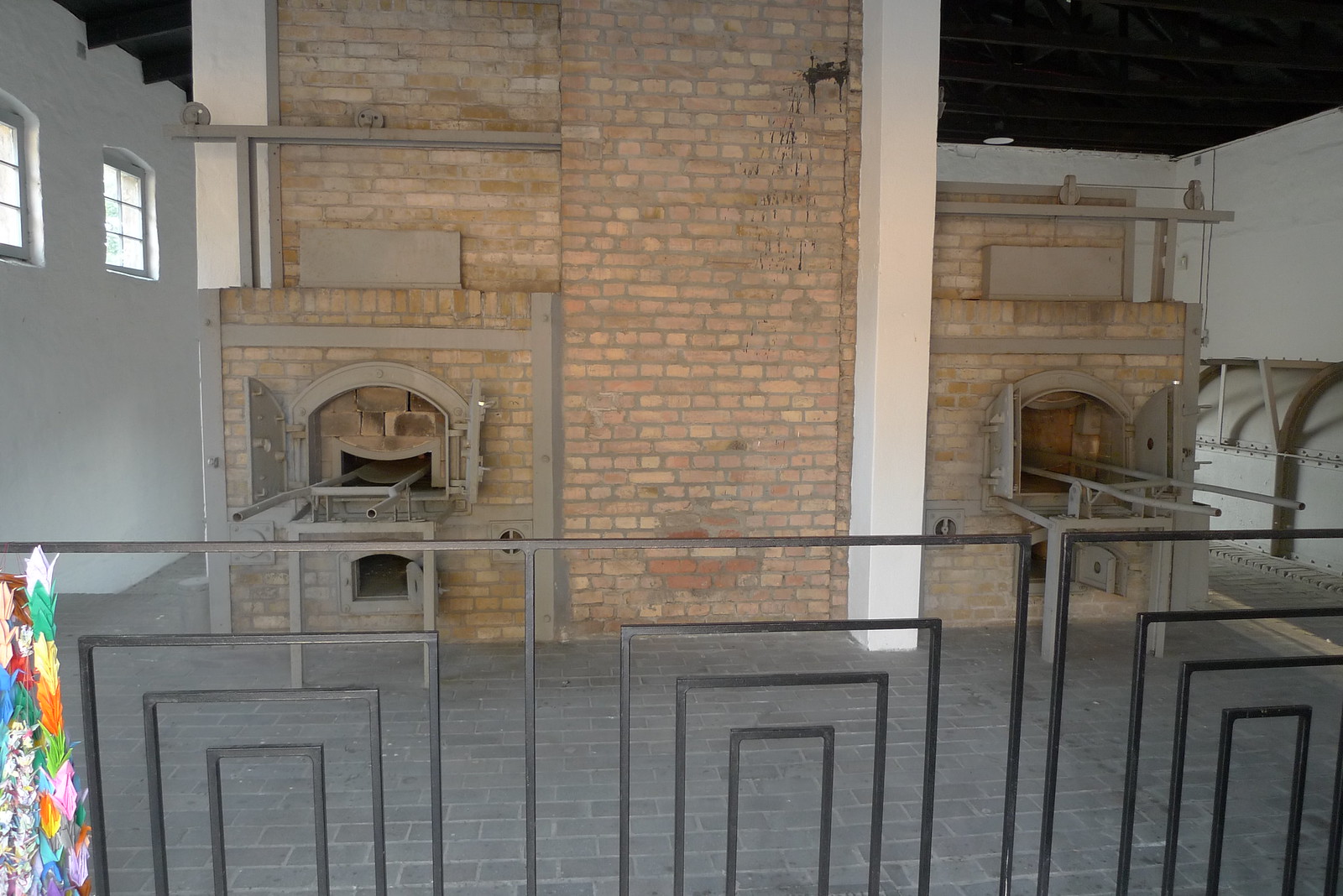The image showcases an interior of a vintage building, possibly a historic crematorium or a large industrial oven. Dominating the scene are two substantial brick structures, akin to kilns or old-style autoclaves, which feature dual chambers with metal slides and dark-gray ironwork. These structures appear designed to burn or heat objects. The foreground contains a black wrought-iron fence with rectangular patterns, adorned with a colorful array of flowers in hues of green, yellow, orange, pink, and blue. Dark gray-bricked flooring spans the area, bordered by white walls on either side. The left wall is fitted with two large windows composed of six small squares in each, while the right wall holds a wooden, metal rack. The room's ceiling is constructed from dark wood and metal, emphasizing the historical and somewhat industrial atmosphere of the space.